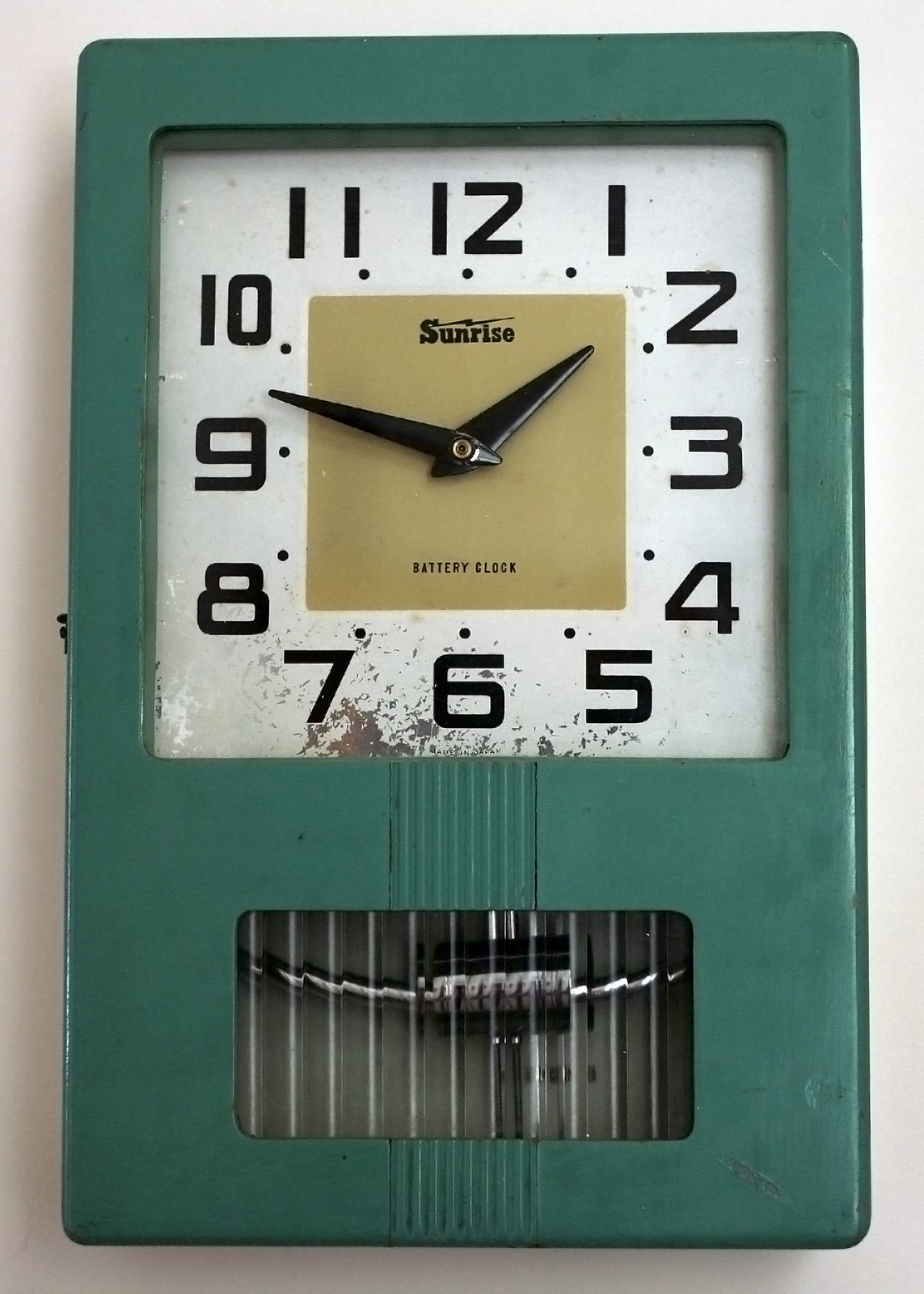This is an image of an old-fashioned, vertical rectangular battery clock made of teal green metal. The clock features a white face with very large black numbers and thick black hands showing the time at 1:47. Positioned in the middle of the clock face is a tan or gold square that prominently displays the word "Sunrise" in black letters, along with the designation "Battery Clock." At the bottom of the clock, there is a clear panel revealing a silver component with metal wires extending from the left to right sides, all resting on a white surface. The clock's surroundings are a gray background, and the overall design includes a bumpy, corrugated texture along the bottom portion of the clock, enhancing its vintage aesthetic.